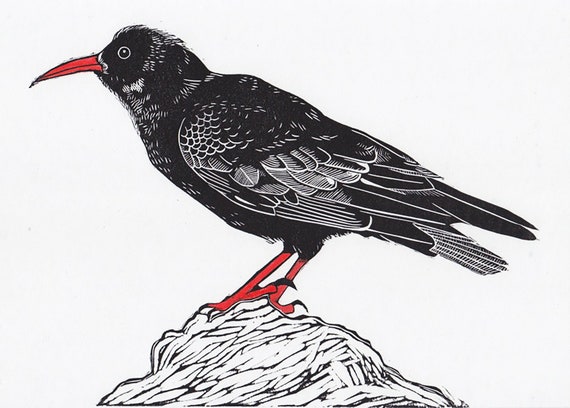The illustration features a medium-sized bird depicted from the left side, standing on a primarily white rock with black outlining. The bird's body is predominantly black, accented by white and gray feathers. It has a striking red beak, red feet, and black claws. The bird's eye is black with a white highlight. The artwork's background is entirely white, creating a stark contrast with the bird and the rock, emphasizing the details of the bird's red and black features and the intricate lines on the rock that give it depth.